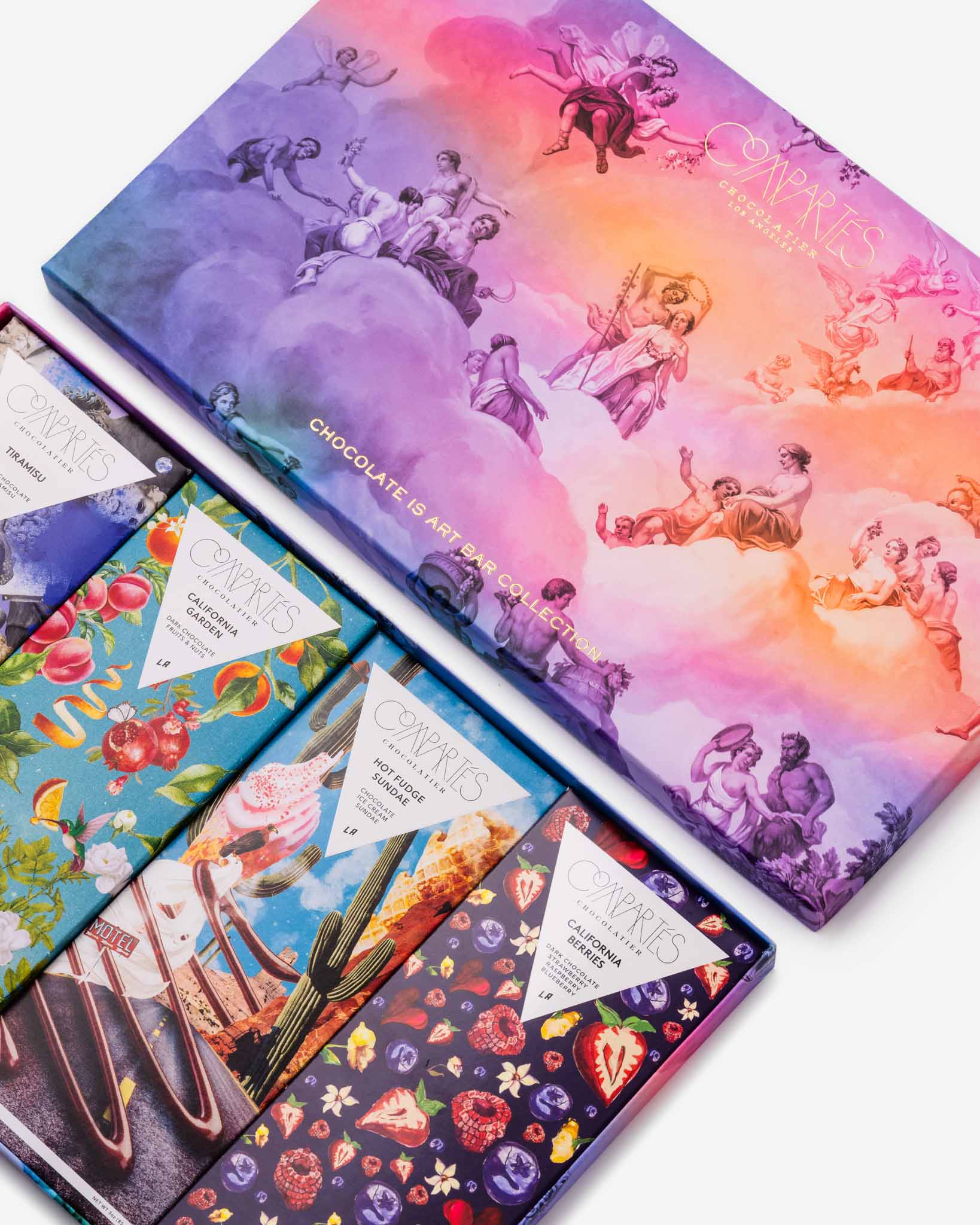The photograph, in portrait orientation, showcases a sophisticated boxed set of Compartes chocolates. The box itself is angled from top left to bottom right, partially cropped at the left and bottom edges. Resting on the same angle above it is the lid of the box, featuring an elaborate design inspired by Michelangelo's "The Creation of Adam," with Greek mythological figures and angels elegantly floating among pink, purple, and orange billowing clouds. The artwork exudes a heavenly and ethereal essence.

Centralized at the top of the lid is the logo "Compartes," followed by "Chocolatier" and "Los Angeles" underneath. Inscribed in gold at the bottom of the cover is the phrase "Chocolate is Art Bar Collection," emphasizing the luxurious nature of the chocolates.

Inside the main box are four meticulously wrapped chocolate bars, lined up vertically. Each bar has a unique, vibrant design: 

1. Tiramisu - illustrated with intricate patterns.
2. California Garden - depicting a scenic road with desert cacti and mountainous backgrounds.
3. Hot Fudge Sundae - featuring indulgent dessert imagery.
4. California Berries - adorned with various berries set against a black background.

Each wrapper includes a white triangle housing the Compartes logo, followed by the flavor designation in black text. The photograph captures the detailed luxury and artistic flair of the chocolate collection, embodying the essence of Photographic Representationalism and Product Photography.